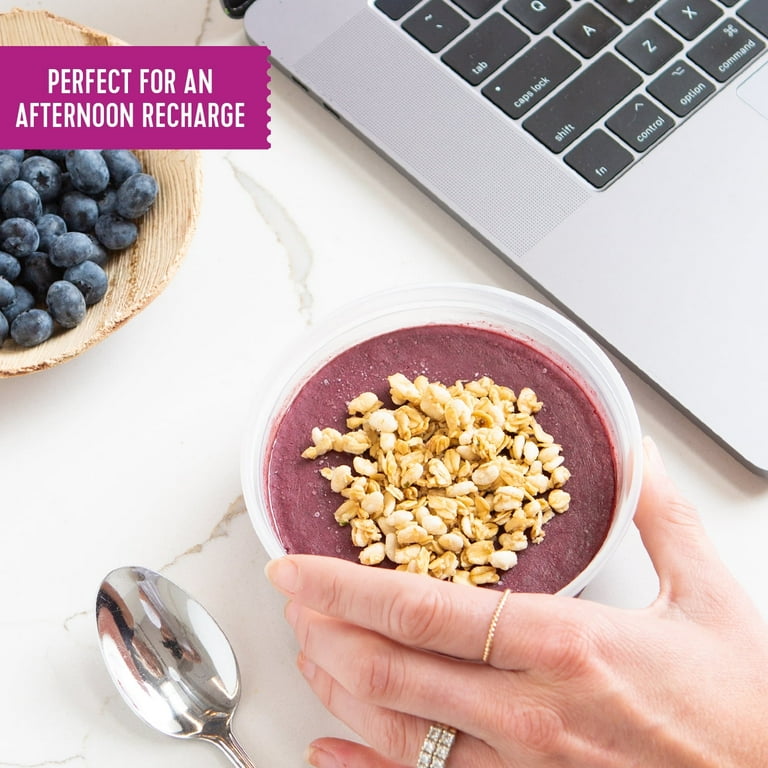The image depicts an indoor setting featuring a vibrant and appetizing scene centered around an acai bowl. The acai bowl, presented in a clear plastic container, has a rich rosy-purple base and is topped with blueberries and a sprinkling of brown granola, nuts, or oats. To the top-left corner of the bowl is a corner of a white ceramic bowl that holds more blueberries, partially covered by a magenta or purple ribbon. The ribbon has an inscription in all capital white sans serif font that reads "PERFECT FOR AN AFTERNOON RECHARGE." The scene is set on a white table, which has subtle browny-grey marks. In the upper right of the image, the silver corner of a MacBook is visible, showing part of the black keyboard with letters Q, A, Z, and X discernible. The bowl is being held by a white female hand adorned with two rings: a diamond ring on the wedding finger and a small gold band on the index finger. The bottom of the image shows the top part of a spoon.